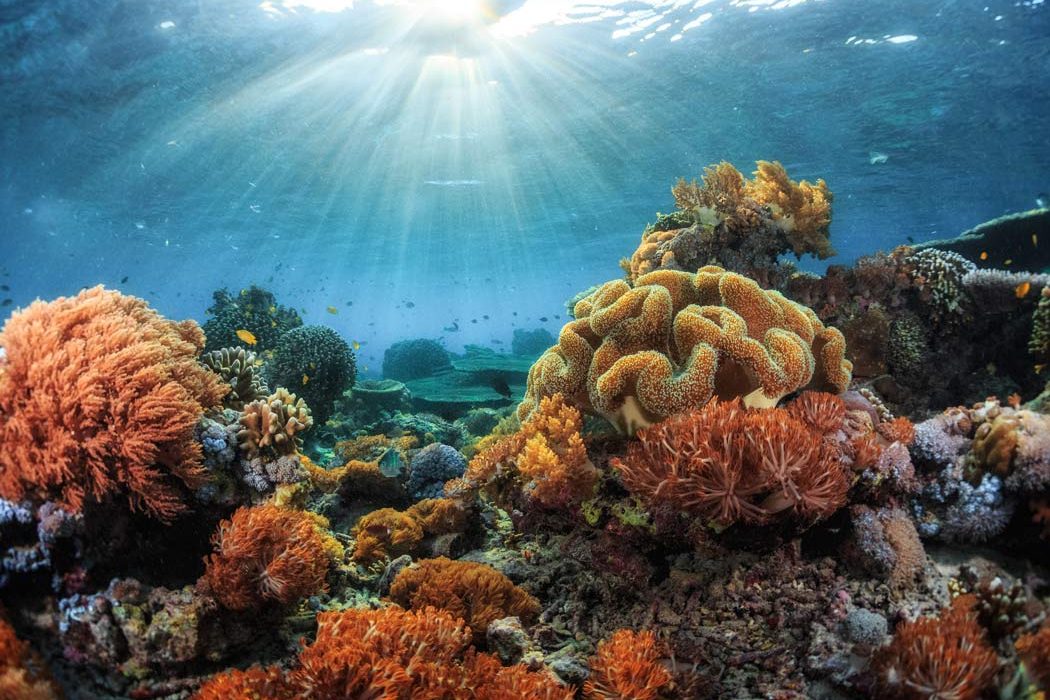This underwater image showcases a vibrant, sun-dappled seascape with a rich variety of marine life and plant structures. At the top of the picture, sunlight penetrates the water's surface, creating mesmerizing beams of light that fan out in various directions. The middle section of the image is dominated by a beautiful, deep blue expanse of water, where small fish silhouettes can be seen swimming in the distance.

Anchoring the scene are the bottom and foreground, teeming with an array of coral and plant life. There are ropey, worm-like yellowish-orange plants snaking together, contrasting with spiny orange structures and patches of white coral. Amidst these are vibrantly colored elements, including purple and blue small coral plants, as well as orange and brownish-orangish coral formations. Rocks pepper the seabed, some adorned with either coral or yellowish plants. A mixture of reddish-whitish plants adds further variety to the scene.

In the center of the image, focal points include yellow fish and a gray fish swimming toward the viewer between two rocks. Above them, the light beams create a beautiful sunray pattern, emphasizing the serene and ethereal quality of the underwater world. The overall scene is a captivating snapshot of marine biodiversity, with a backdrop of greenish bushes and large rock formations enhancing the sense of depth and complexity in this aquatic habitat.